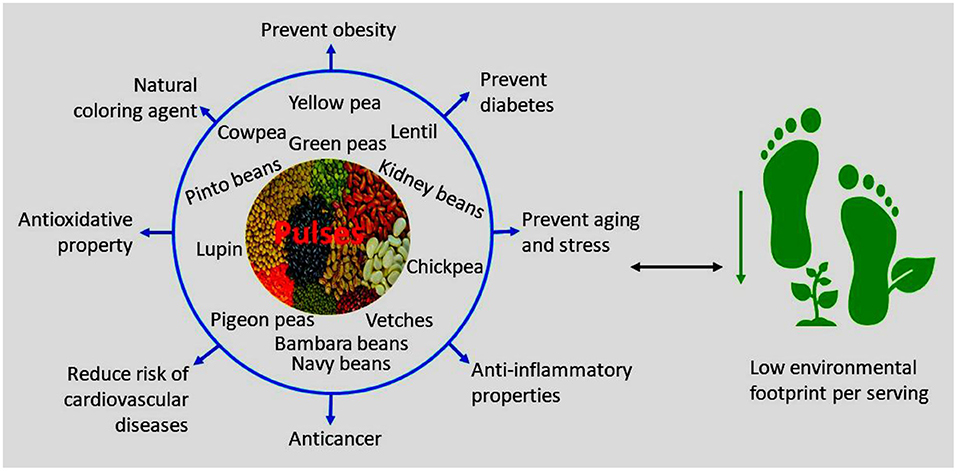This detailed infographic highlights the benefits of legumes and pulses. On the right side, it features two cartoon-drawn bare feet surrounded by greenery, symbolizing a low environmental footprint per serving. Moving to the left, there's a central blue circle, designed with arrows extending outward like a clock face. Each arrow points to a specific health benefit: preventing obesity, preventing diabetes, preventing aging and stress, possessing anti-inflammatory properties, anti-cancer effects, reducing the risk of cardiovascular diseases, having anti-oxidative properties, and serving as a natural coloring agent.

Inside the blue circle, a variety of legumes, peas, and beans are listed randomly. At the core of the circle, a photo of beans is prominently displayed with the word "pulses" written in bold red lettering across it. The comprehensive design effectively communicates both the environmental and extensive health benefits of incorporating legumes into your diet.